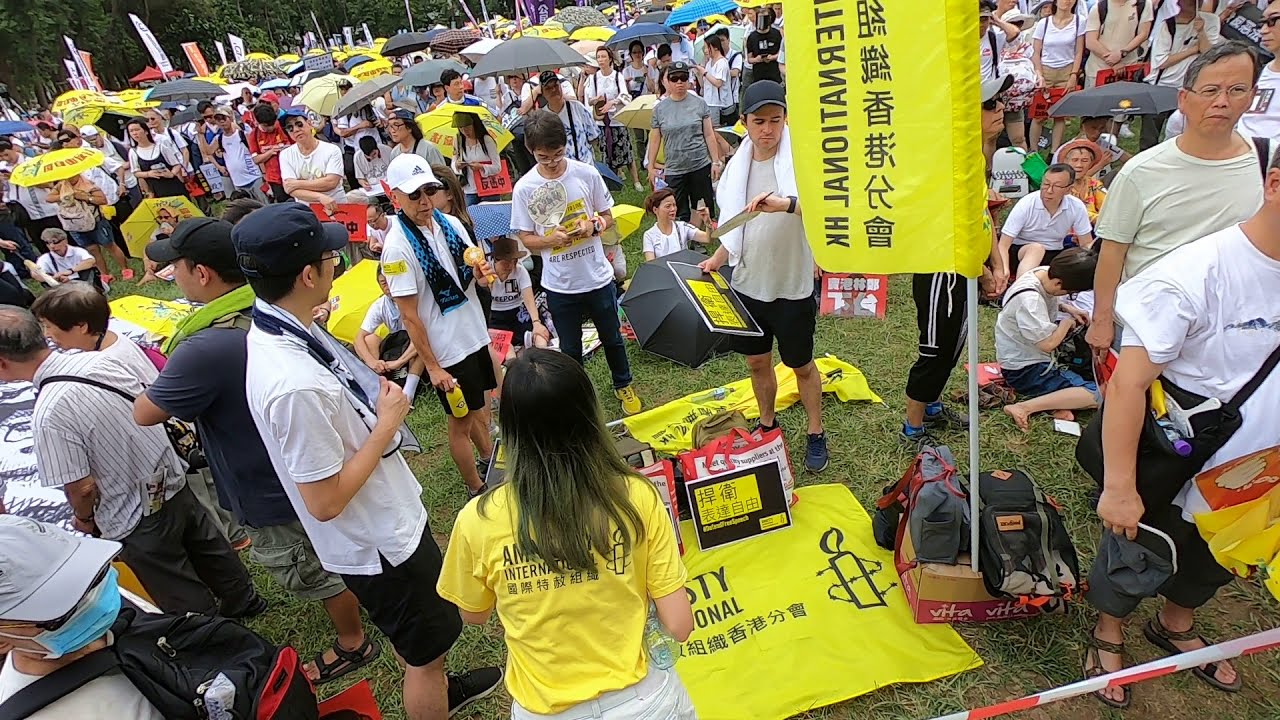The photo shows a large gathering of people, likely in an Asian country or involving a significant number of Asian refugees, taken outside what appears to be a refugee camp or rally organized by Amnesty International. Central to the scene is a person at the front wearing an Amnesty International shirt, and a flag with the organization's name is visibly waving nearby. On the ground, there is a towel with the same text, suggesting a setup possibly intended to promote Amnesty International’s cause or engage attendees. The crowd, predominantly facing the camera, features numerous individuals holding yellow, black, gray, and blue umbrellas, creating a striking visual pattern. Many people are holding yellow signs with Asian characters, further indicating the probable location and cultural context of the event. The scene conveys an atmosphere of solidarity and advocacy among a diverse assembly of people.